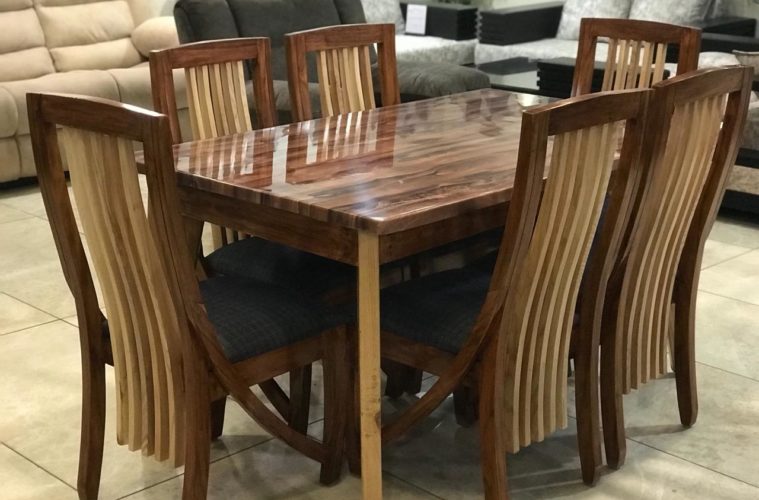This detailed photograph, likely taken inside a furniture store or intended as a stock image for kitchen furniture, features a striking wooden table set placed diagonally on a cream-colored ceramic tile floor. Central to the image is a glossy, rectangular dark brown wooden table, highlighted by its laminated and polished surface. The table is accompanied by six unique chairs: two positioned lengthwise on either side and one at each end. These chairs boast a distinctive design with their backrests extending down and curving to the front, traditional four-legged structure. The chair frames are dark brown wood, contrasting with the light tan or beechwood slats on the backrests that add intricate detail. The deep blue cushioned seats add a pop of color against the otherwise neutral shades of brown, tan, black, gray, and white throughout the image. In the background, occupying the top portion of the photo, are various couches and a recliner-style chair, further suggesting the setting is within a furniture showroom.